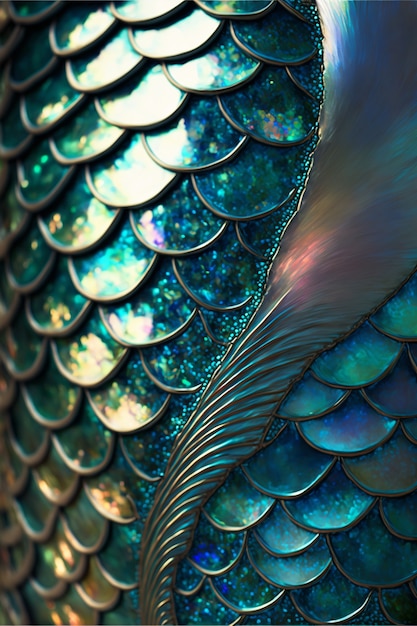This image is a close-up of a colorful, intricate piece of jewelry, likely a glass peacock or similar artistic creation. The objects within the image are rounded, circular segments with metal bands surrounding vibrant pieces of colored glass. These segments overlap and are predominantly colored in shades of green, blue, and turquoise with multicolored spots including light blue and orange. The jewelry exhibits a gradient from the center to the sides: the right side shows clearer, in-focus segments, while the left side is slightly blurred. A vertical element extends from the bottom to the top right, perhaps a large leaf or a structural component, featuring ridges at the bottom and becoming wider as it ascends. Reflective light adds a shimmering effect to the glass, especially prominent on the left side. The background is entirely obscured, focusing attention solely on the elaborate detailing of this artistic piece.